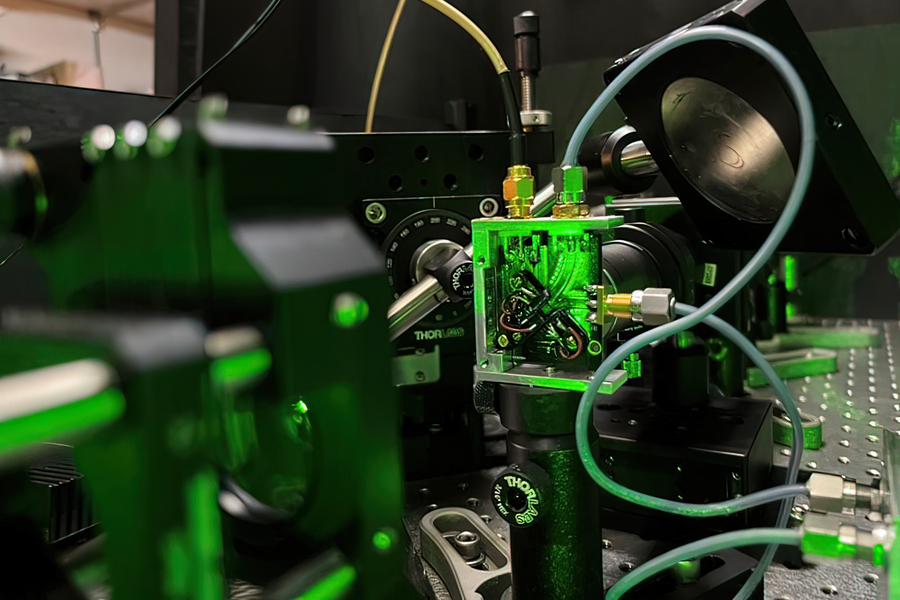The image displays a close-up of a modern, new-looking machine with a silver, metallic color and black accents on various parts. Prominently featured in the center is a small, see-through green square emitting green light, likely reflecting internal lighting. This green square is attached to a stand adorned with the letters "T-H-O-R-L-A-R-S". Several wires in different colors, including gray, yellow, blue, and black with gold, connect to various parts of the machine. The blue wire runs to devices located on both the left and right sides of the machine. The intricate setup includes gauges, bolts, a large black box with a protruding silver rod, and a slanted plate with silver in the middle. The entire apparatus is situated in a room with black walls and no visible natural light, suggesting an indoor experimental environment.